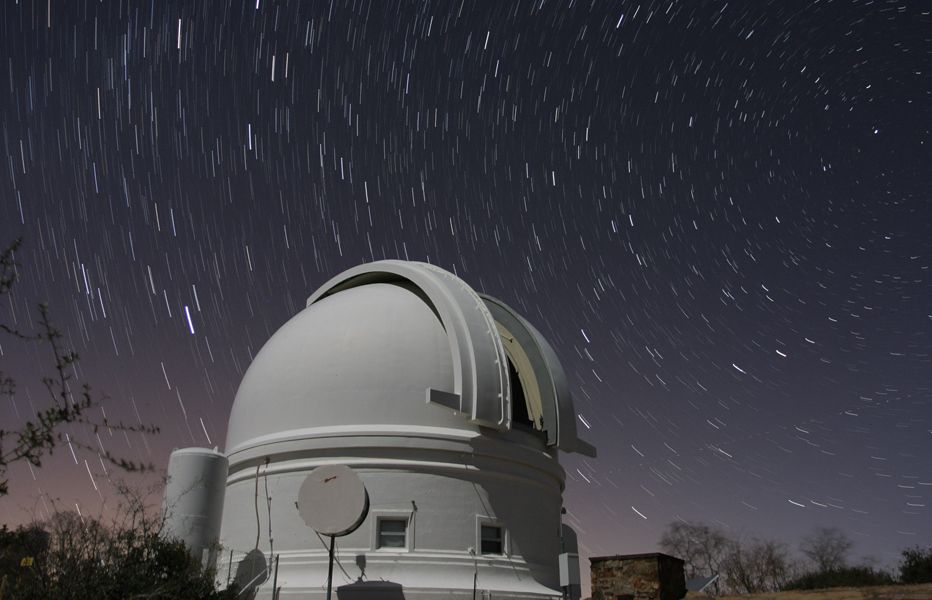The image depicts a rectangular photograph approximately six inches wide by four inches high, capturing an observatory set against a hyper-realistic night sky, likely enhanced with filters for dramatic effect. The stars, initially appearing as small dots on the right side of the sky, progressively elongate and swirl in a circular motion toward the left, suggesting a time-lapse or long exposure technique that captures the Earth's rotation. The night sky is a blend of dark hues with hints of pinks and blues, further enriching its surreal appearance. In the background, there are bare treetops indicating a winter setting, while the lower left corner reveals more treetops, and the lower right corner includes a small brick chimney.

The focal point of the image is a large gray domed building at the center bottom, identifiable as an observatory due to its sliding top presumably designed for a telescope, though it appears closed. This building features a rotunda around the top and a few windows near the base. Adjacent to this main structure is a smaller stone brick building and a cylindrical tower, adding layers to the composition. The entire scene exudes a serene yet dynamic atmosphere, with the swirling star trails emphasizing the observatory’s purpose of watching the cosmos.